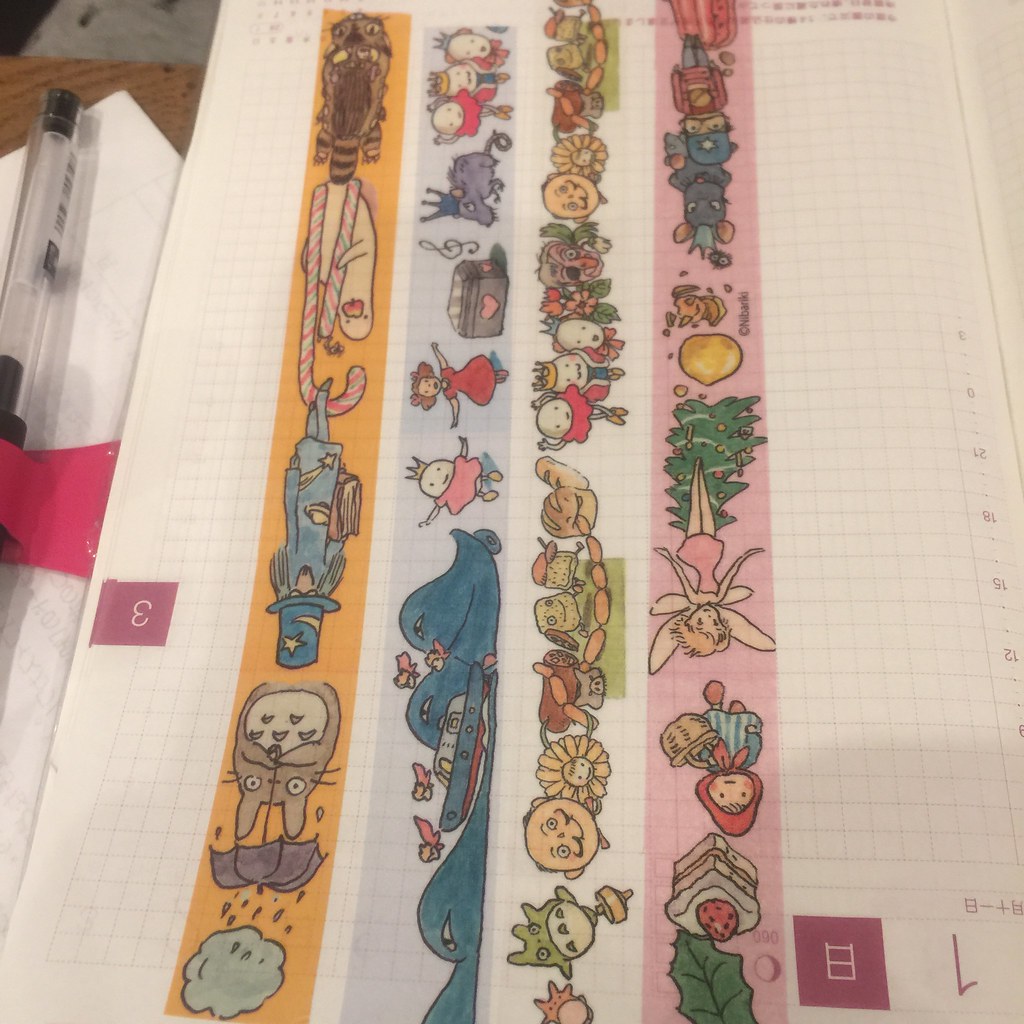The image features a Japanese notebook placed upside down on a brown table, partially visible in the upper left corner. The open notebook reveals a piece of white graph paper with numbers and fine lines, arranged in a clean, organized grid. Centered on the paper are four long strips, possibly temporary tattoos, each adorned with whimsical, child-friendly cartoons on varying colored backgrounds including pink, purple, yellow, white, orange, and light blue. The strips display a delightful array of characters and scenes: a rabbit with an umbrella under a shower of rain, a playful parrot perched on a candy cane, an endearing owl, animated figures near an oven, whimsical whales near a ship, a fairy by a Christmas tree, a cheerful mouse, and a delectable piece of strawberry cheesecake. These vibrant strips capture the imagination with their charming and colorful designs. A black pen lies off to the left of the notebook, and Japanese lettering is faintly visible on the cover.